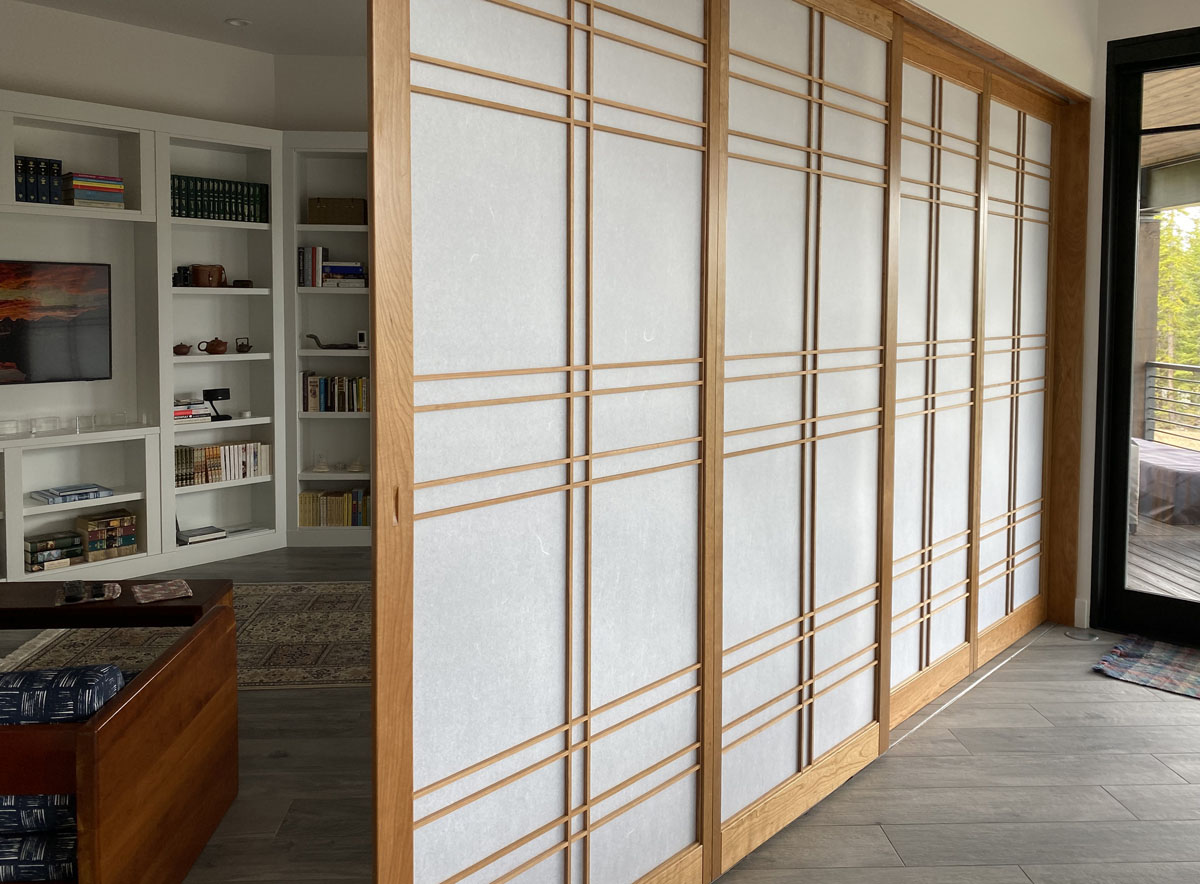This photograph captures an indoor entryway leading to an entertainment room or library, characterized by a harmonious blend of utility and design. The focal point of the image is the series of sliding Japanese screens, framed in light wood with rice paper inserts, that can be moved to open or close certain parts of the room. These screens, reminiscent of traditional tatami home features, create a flexible space within the white-walled interior embellished with vertical wood accents.

To the right of the screens, a steel door with a clear glass panel reveals a daytime outdoor scene, including a deck with a black railing, a small beige table, and a backdrop of trees. Adjacent to the door, a checkered mat in blue, pink, green, cyan, and beige lies on a faux wood beige floor.

Inside, the room features a wrap-around white bookcase organized with numerous books in varying colors. At its center, a photo or LCD TV is mounted above neatly stacked books. A dark wood piece of furniture with blue couch cushions and multicolored napkins is positioned towards the bookcase's edge, adding to the room's cozy aesthetic. The space is pulled together by an embroidered rug at the center, and a table in the lower left corner with a board game, hinting at the room's versatile use for leisure and entertainment.